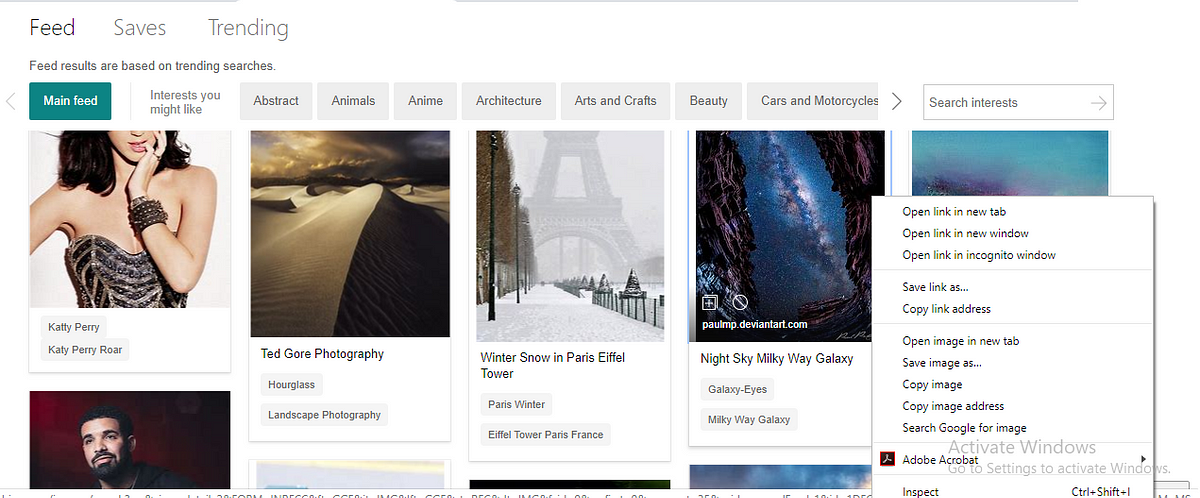This is a screenshot from an unidentified website, featuring a detailed layout of its feed page. At the very top, there are three navigation options labeled 'Feed,' 'Saves,' and 'Trending,' with 'Feed' being the currently selected tab.

Directly beneath this main navigation bar, it is indicated that "feed results are based on trending searches." Further down, another navigation bar offers various categories for selection. These categories include 'Main Feed,' 'Interests You May Like,' 'Abstract,' 'Animals,' 'Anime,' 'Architecture,' 'Arts and Crafts,' 'Beauty,' and 'Cars and Motorcycles.' The 'Main Feed' category is currently selected, highlighted with a dark turquoise color.

In the 'Main Feed' section, there are several articles displayed, each accompanied by a related photo. Notable articles include:
- "Katy Perry"
- "Ted Gore Photography" tagged with 'hourglass' and 'landscape photography'
- "Winter Snow in Paris, Eiffel Tower" tagged with 'Paris winter,' 'Eiffel Tower,' 'Paris, France'
- "Night Sky, Milky Way Galaxy" tagged with 'Milky Way Galaxy' and 'Galaxy Eyes'

Additionally, someone has right-clicked on the page to reveal the typical context menu options available in the Google Chrome web browser. These options include 'Open link in new tab,' 'Open link in new window,' 'Open link in incognito window,' 'Save link as,' 'Copy link address,' 'Open image in new tab,' 'Save image as,' 'Copy image,' 'Copy image address,' 'Search Google for image,' 'Adobe Acrobat,' and 'Inspect.'